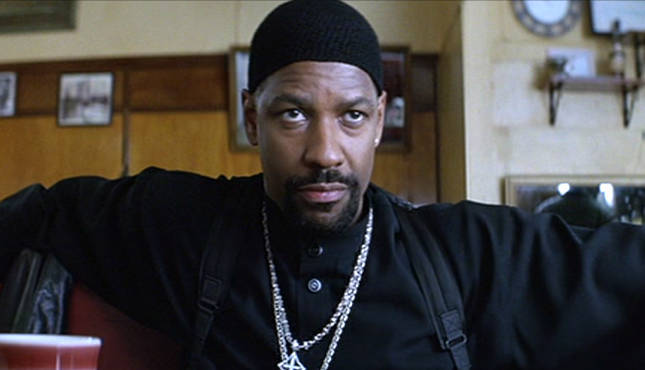This is a color photograph featuring Denzel Washington in a movie still from the film "Training Day." He portrays an undercover police officer, emanating a serious and menacing presence. Washington, an African-American male, is dressed entirely in black, including a long-sleeve shirt, a tight black beanie, and the visible straps of a shoulder holster. Around his neck, he sports two heavy, white gold or silver chains. He is seated in a diner, characterized by its walls adorned with framed photographs, plates, mirrors, and shelves. Washington is seated in a red chair or sofa, with a red cup in front of him, and he is gazing intently at someone opposite him. The setting and his posture enhance the intensity of the scene.